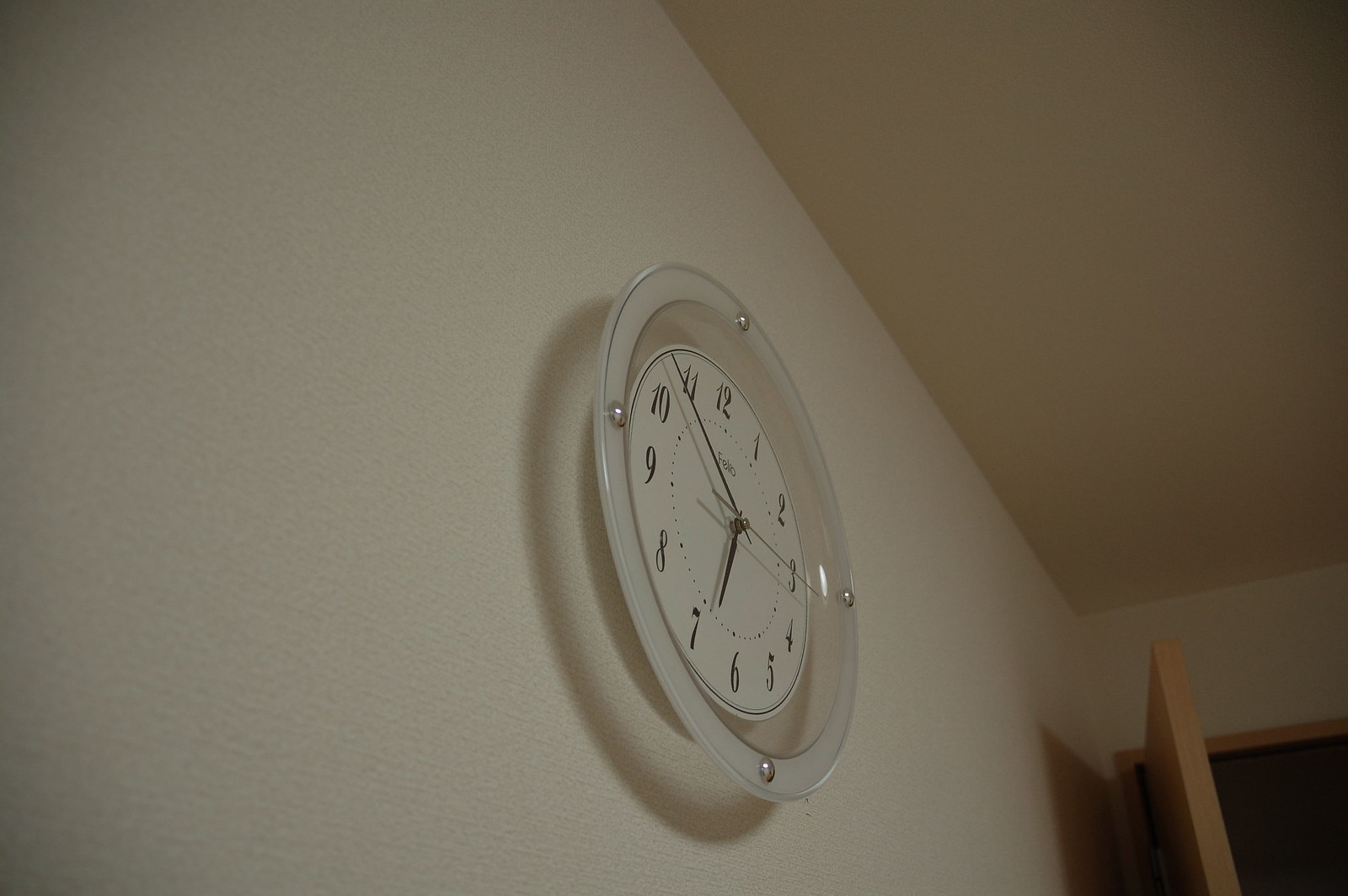This photograph captures a wall-mounted clock set against a pristine white wall. To the right side of the image, the corner of the room is visible, seamlessly connecting the white ceiling and walls. Adjacent to this corner, a brown door with matching brown trim stands ajar, casting a subtle shadow on the wall. The clock itself features a clear base with a white outer ring, adorned with four sleek silver buttons. The time displayed is approximately 6:52:15, indicated by the visible minute, hour, and second hands.